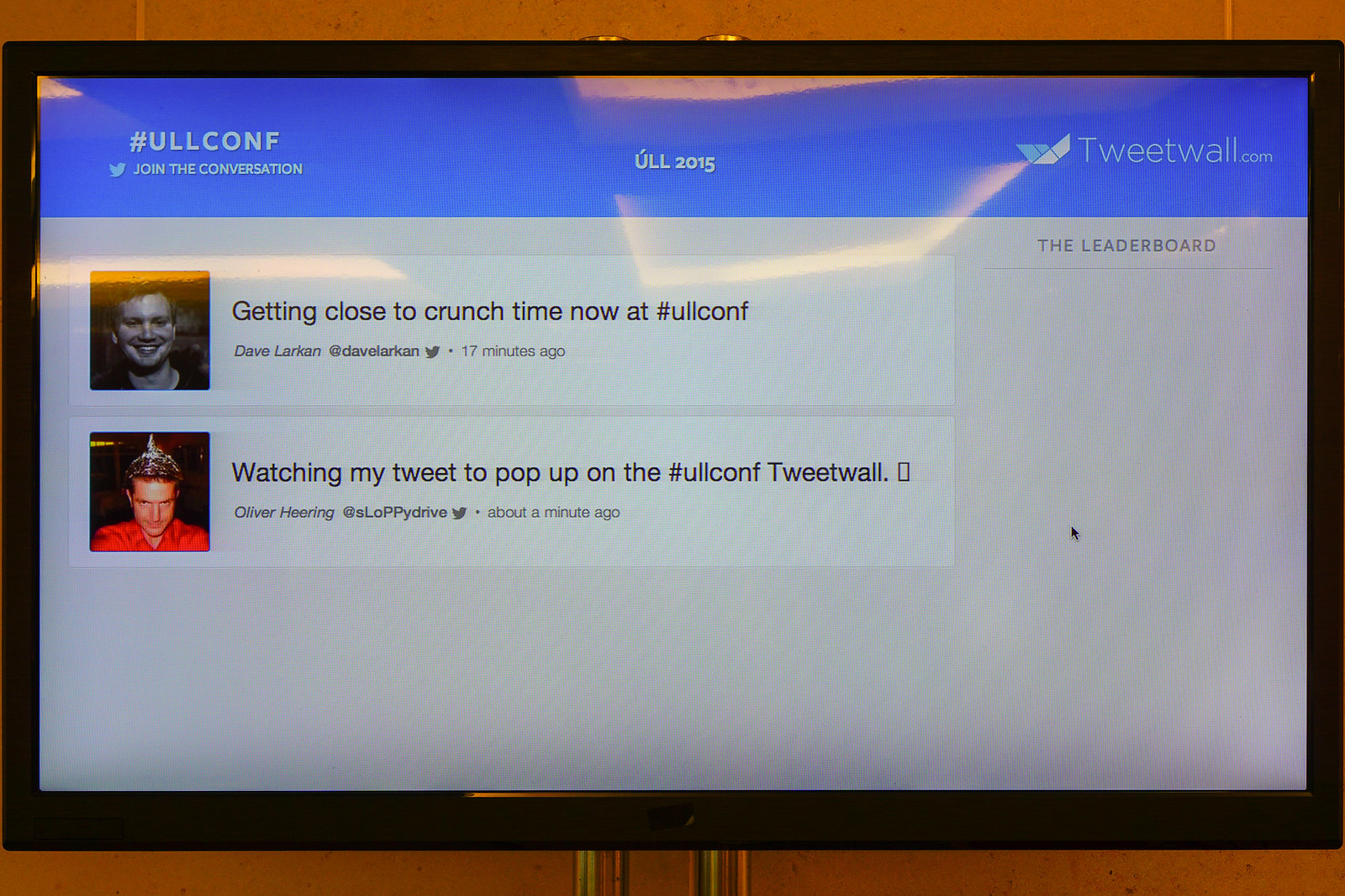The image shows a black-colored tablet displaying a page from Twitter against a brown or orange background. At the top of the page in white letters on a light blue background is "#ULLCONF Join the conversation" followed by a blue Twitter symbol. Below that, on an all-blue background, the text "ULL 2015" and "tweetwall.com" are displayed alongside a folded blue Twitter symbol. To the right of the screen is a gray section titled "Leaderboard" with a black pointer indicating a mouse cursor.

One prominent tweet displayed on a white background features a black and white image of a man and reads: "Getting close to crunch time now at #ULLCONF Dave Larkin @davelarkin" with a timestamp of "17 minutes ago" in gray letters. Below this, another tweet with a photo of a man in a red shirt against a dark background says: "Watch my tweet pop up on the #ULLCONF tweetwall" from Oliver Heiring (@sloppydrive), posted "about a minute ago" in black letters.

The overall scene resembles a projected display or overhead projector setup, possibly used in a teaching or presentation context. The setup has black framing surrounded by a brown background, suggesting it might be placed against a brown wall.